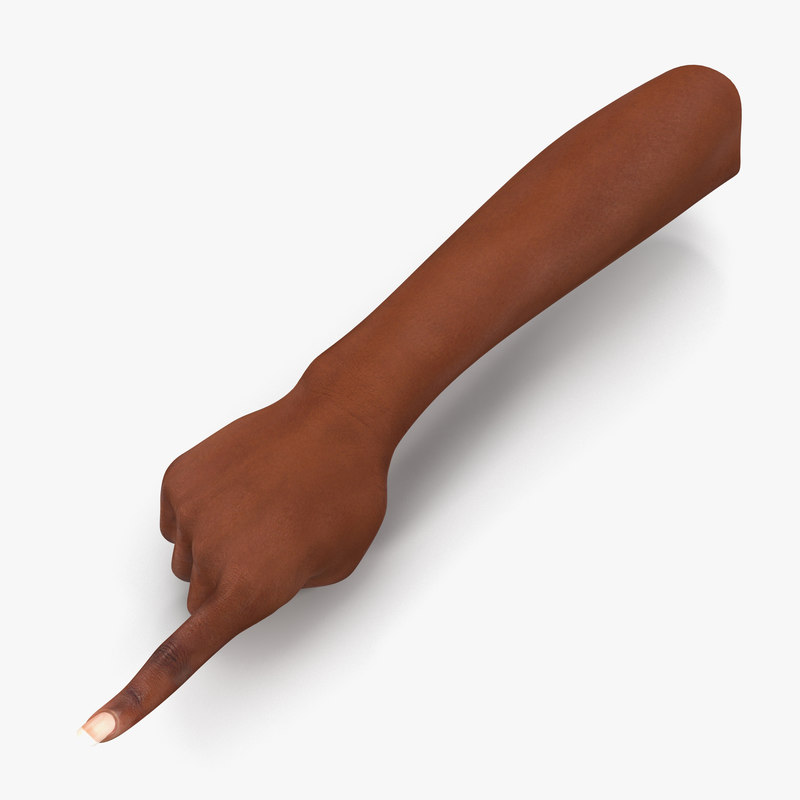The image depicts a dark brown, smooth-skinned arm that appears either computer-generated or part of a manipulated photograph. The arm is cut off just before the elbow and is positioned diagonally against a solid white background, extending from the upper right-hand corner to the lower left-hand corner. The hand is relaxed, with all fingers pointing down except for the index finger, which distinctly points towards the lower left corner. The index finger features a short nail with a French tip manicure. The arm's surface is unblemished and free of scars or wrinkles, and a shadow of the arm can be seen directly below its path.